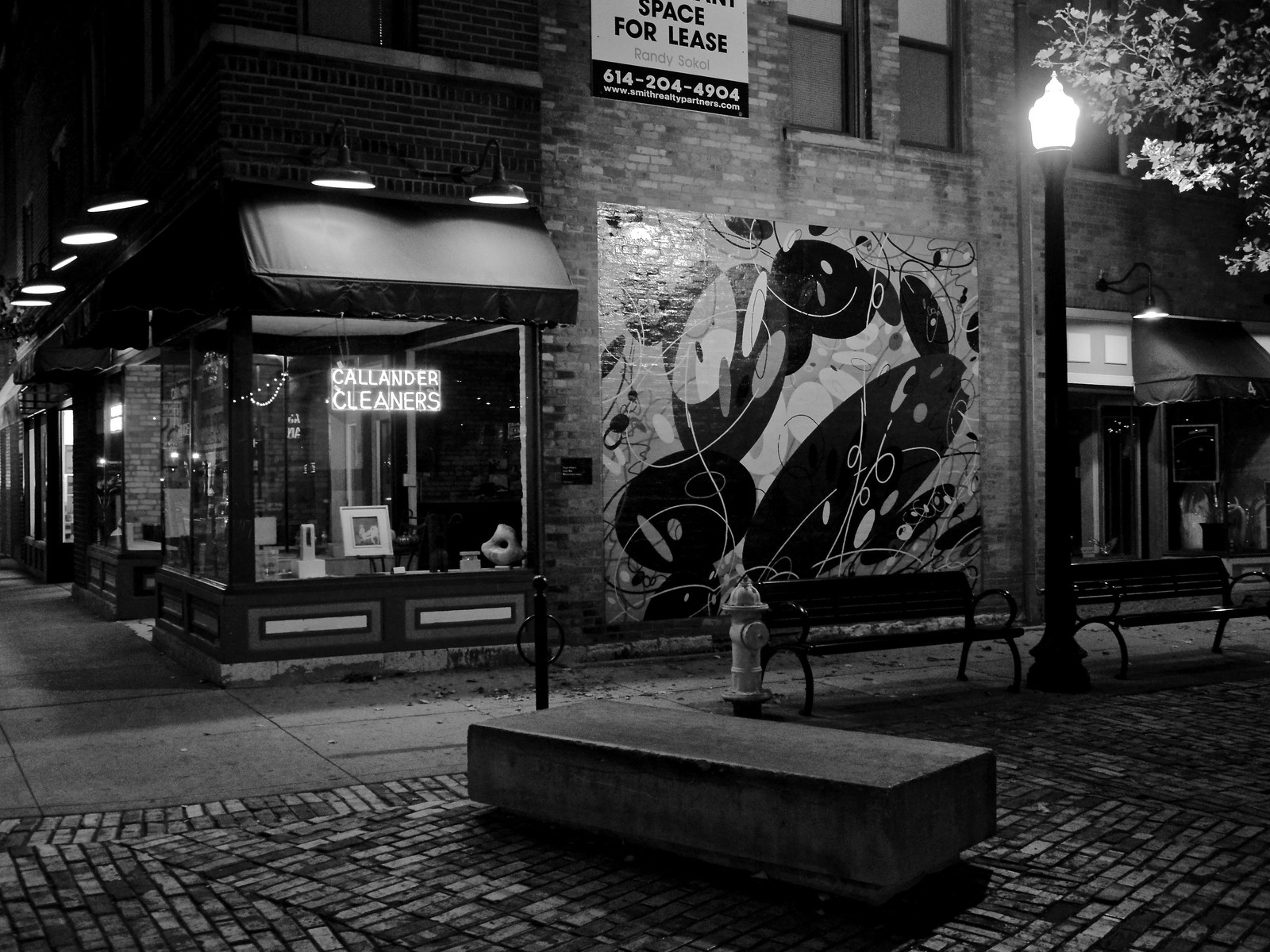The black and white photo, taken at night, captures an outdoor scene featuring a street corner with an urban square. The square is paved with brick laid in various shapes and includes park benches and a fire hydrant. On one side of the square stands a brick building, adorned with a mural of intricate black and white shapes. This building displays a sign reading "Space for Lease" along with a phone number. Adjacent to this building, another storefront can be seen with large, illuminated glass windows bearing the name "Colander Cleaners." Additionally, a notable sculptural object or artistic installation is situated near the sidewalk, adding to the urban aesthetic of the scene. The area appears deserted, emphasizing the stillness of the night.